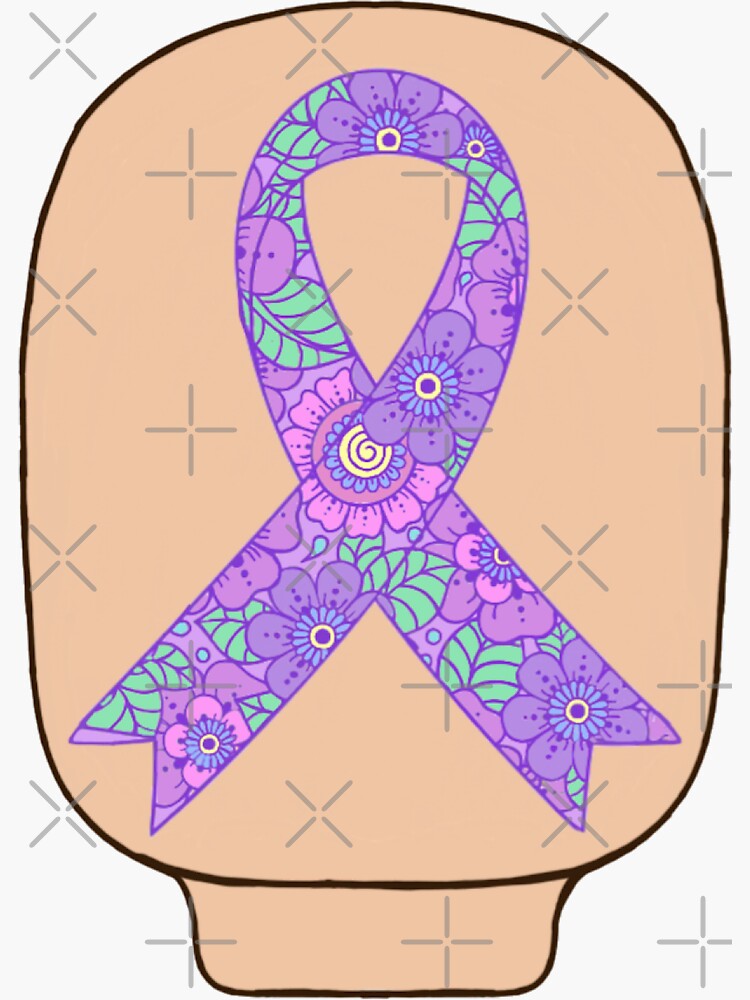This image depicts a highly stylized ribbon meticulously adorned with an array of flowers and leaves in vibrant hues of purple, green, pink, blue, and yellow. The ribbon is prominently positioned in the center and features an intricate, 60s style floral pattern. It appears to be set against a layered background, starting with a yellow area outlined clearly, behind which lies a stark white surface. This white background is intricately patterned with repeating gray Xs and crosses, symmetrically placed across the entire image. Interestingly, the overall shape and positioning of the ribbon suggest a resemblance to a headrest with an oval top, tapering down to a neck-like extension. The image evokes the form of a cancer ribbon, symbolically folded and vividly expressive against its thoughtfully detailed backdrops.